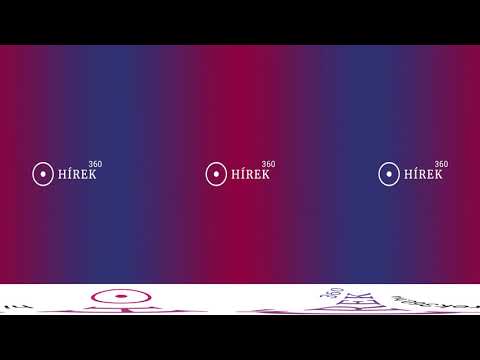The image is a detailed and stylized graphic design in a landscape orientation, featuring a repeated logo three times across the center. This logo includes the text "HIREC 360" in white lettering, each accompanied by a bullseye target icon. The background displays a series of red and blue vertical gradient stripes, giving the appearance of repeating color columns. Across the top and bottom of the image, there are thick black horizontal strips. The bottom strip includes stretched-out text, primarily showing the number "360" alongside partially visible letters in pink and black, on a white background. The image combines photography with graphic design elements and employs specialized filters for an intricate, visually compelling composition.